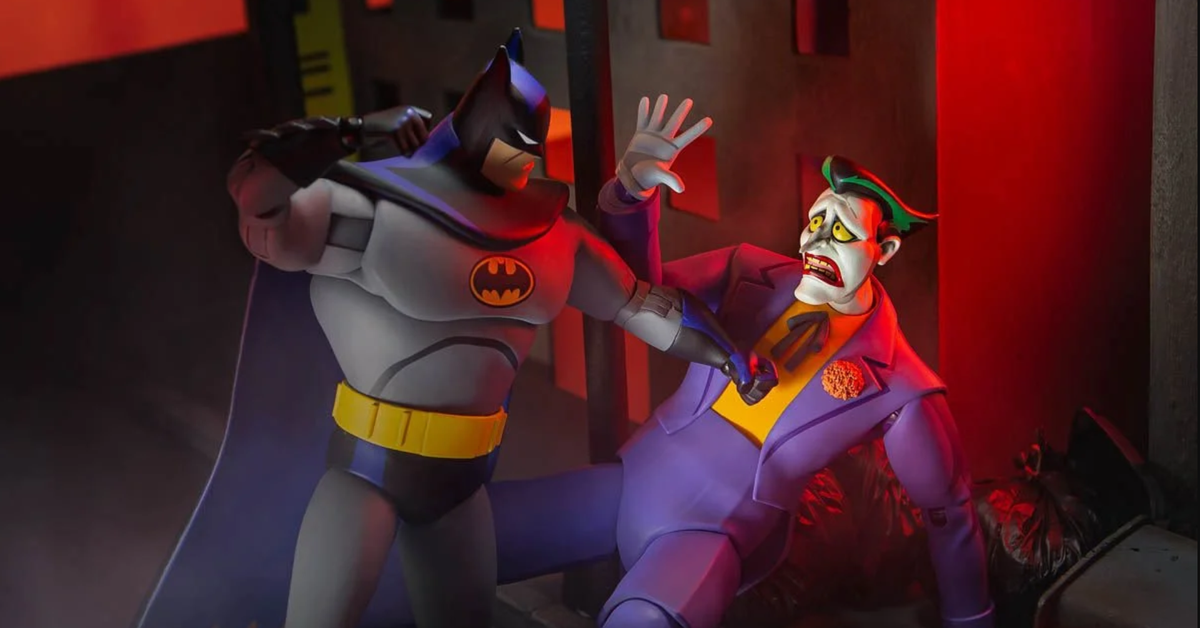In this detailed scene from an animated movie, Batman and Joker, rendered in a clay-like, plastic texture, confront each other in a dark, dramatic alleyway. Batman stands on the left, his imposing figure draped in a gray suit with black boots, underwear, gloves, and a black cowl that features his iconic bat ears. His yellow utility belt stands out against the dark palette. Batman's right arm is cocked back, fist clenched, ready to deliver a powerful punch to the Joker, whose right hand is raised defensively, clad in a white glove.

The Joker, known for his chaotic demeanor, is depicted in his classic villainous attire: a purple suit with a yellow shirt beneath and a large flower on the left lapel. His face is ghostly white, accented with red lipstick, green hair with black streaks, and yellow eyes that convey a mix of fear and defiance. Joker appears to be stumbling backward into a pile of black garbage bags, in a desperate bid to ward off Batman's blow.

The alleyway setting is dark and foreboding, with a red light casting an eerie glow over the scene. Behind the Joker, a fallen trash can and more trash bags add to the atmosphere of disarray. To the right of the scene, a wall and the hint of buildings are visible, contributing to the urban backdrop. A light pole rises between Batman and the Joker, extending off the top of the image, casting the single beam that illuminates this intense confrontation. Overall, the scene captures the high-stakes tension and vivid character details that define their legendary rivalry.